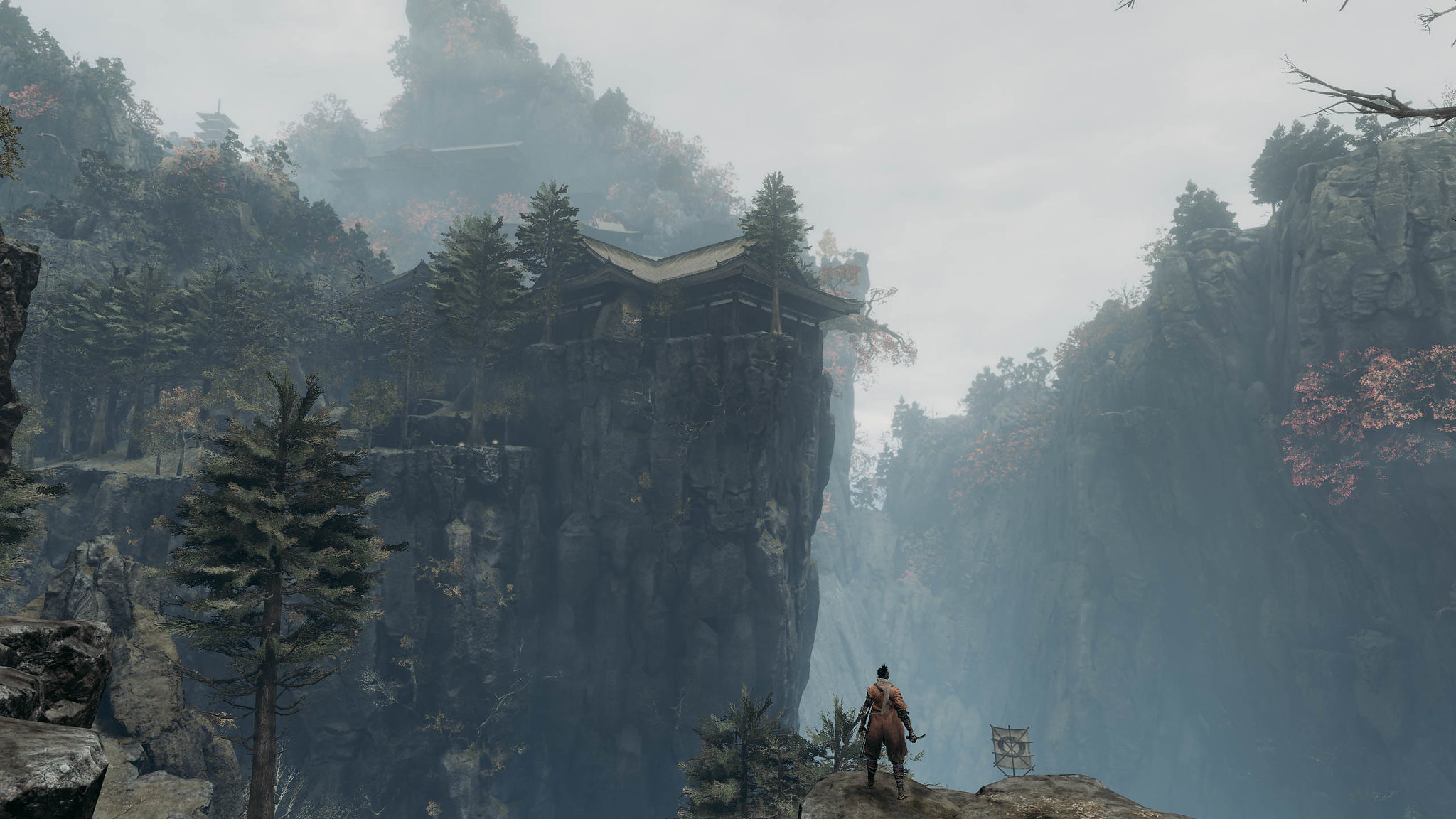The image is a vivid, detailed painting of a natural outdoor scene. Dominating the foreground is a large rock, upon which a man stands, dressed in a tan shirt and pants, holding an unidentified object. Adjacent to him is a small tree, and he gazes into the distance. Behind him, the terrain rises sharply into imposing cliffs adorned with jagged edges in shades of brown and gray. At the top of one of these towering cliffs is a house perched precariously on the edge. Surrounding the cliffs and house are numerous trees and dense foliage typical of a deciduous forest. The sky above is a cloudy gray, adding a somewhat somber yet serene ambiance to the scene. Additionally, there's what appears to be a white flag, perhaps with a pirate motif, positioned on the cliff near the man, enhancing the sense of adventure and contemplation in the painting.